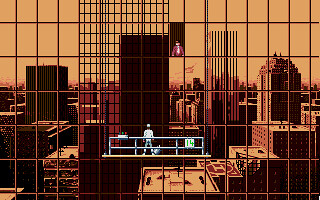This image, resembling a detailed still from a computer-animated video game, depicts a bustling cityscape dominated by a shiny gold skyscraper with reflective windows. The foreground features a window washer standing on a metallic platform, wearing a white uniform, white hat, and blue pants. To his left is a control box with colorful knobs—green, red, black, and purple. The platform is mounted on blue railings, with a white square displaying the number 14 in green on the right side of the railing. Behind the window washer, the city's skyline, with buildings of varying heights, is beautifully mirrored in the skyscraper's glossy facade. Above him, one of the grid-like array of windows is open, revealing a man with dark hair clad in a purple jacket and a white shirt, peering down at the window washer, creating a moment of silent connection amidst the busy urban atmosphere.